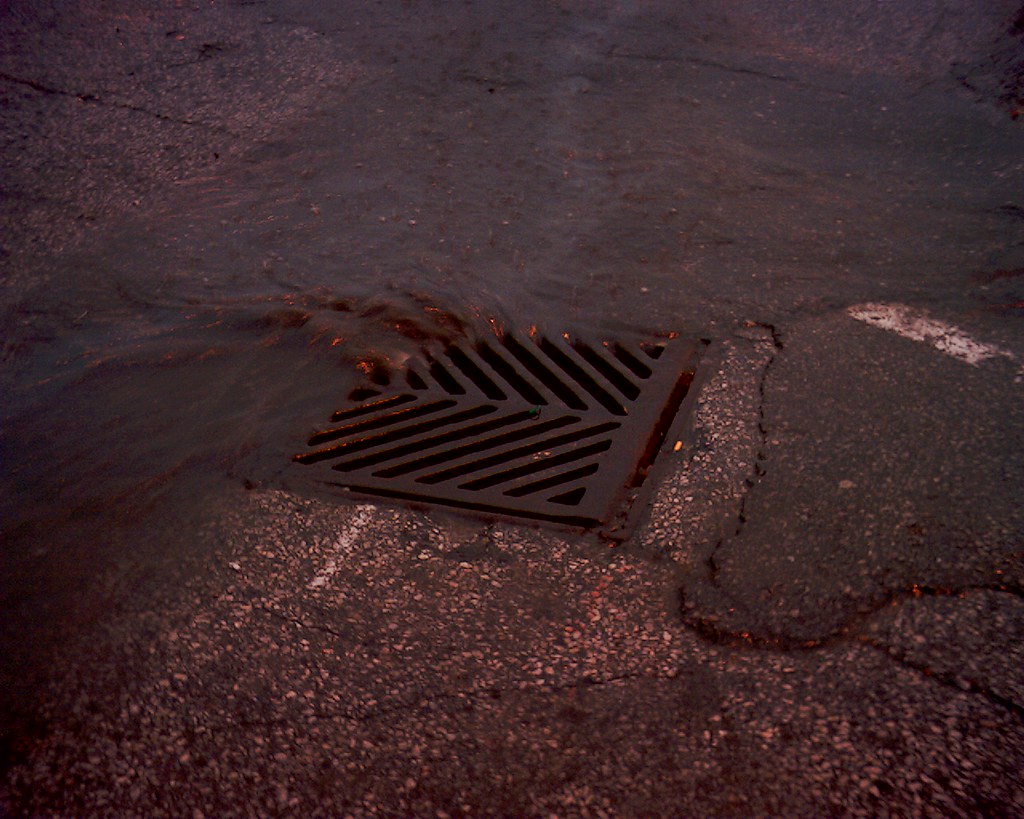This photograph, taken outdoors and set against the backdrop of sunset, captures a worn, cracked, and patched section of an asphalt city street with an emphasis on a central sewer cover. The lighting imbues the scene with a striking pink and brownish-red hue that blends into the darkening surroundings. At the focal point of the image is a square, rusty, brown drain with diagonally cut triangular slats and a central metal rod. Water, tinged with the ambient light giving it a reddish appearance, is rapidly flowing from opposite sides of the roadway towards the sewer cover. Despite this, there appears to be an obstruction, possibly wood, partially blocking the entrance, causing the water to pool and bypass the drain, flowing towards the bottom left of the image. The combination of the sunset's light and the condition of the road sets a compelling and almost eerie mood to the photograph.